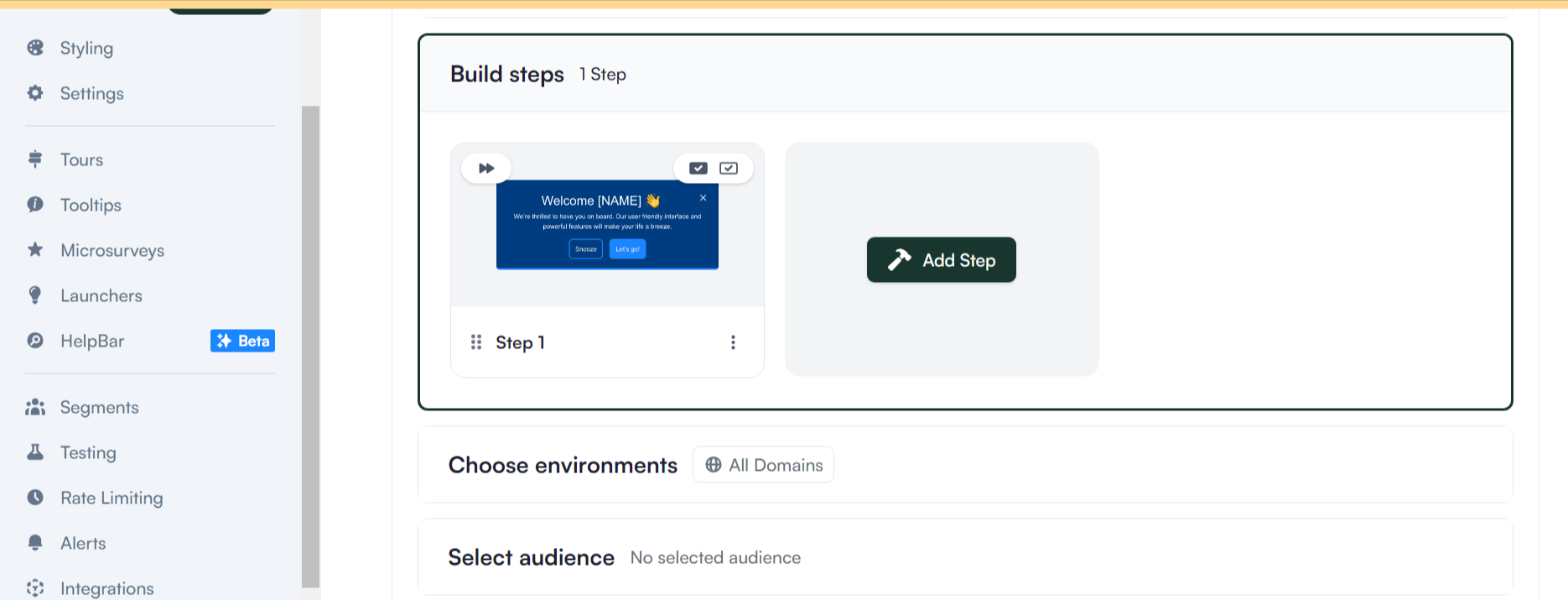This image displays a partial web page from a website. On the left, there is a gray sidebar section featuring various tabs, organized in descending order: "Styling" and "Settings" followed by a faint line, then "Tours", "Tool Pits", "Tool Tips", "Microsurveys", "Launches", and "Help Bar". Adjacent to "Help Bar" is a small "Beta" button. Below another faint line, there are more options: "Segments", "Testing", "Rate Limiting", "Alerts", and "Integrations".

On the right side of the web page, it appears to be a tool for building a website, indicated by a section labeled "Build Steps". This section starts with step one, which is enclosed within a box containing a greeting message "Welcome" followed by the user's name. This box also features a fast-forward icon and two checkboxes, one black and one white. Below this are six vertical dots in a line, representing step one, with three more dots to its right.

Further down, there is a gray section featuring a schematic hammer icon and a central black button with the white text "Add Step". 

Directly beneath this, several white boxes with black text can be seen. The top box is labeled "Choose Environment" and includes a white button with a globe icon and the text "All Domains". Below it is another box titled "Select Audience", with the message "No selected audience" indicated within.